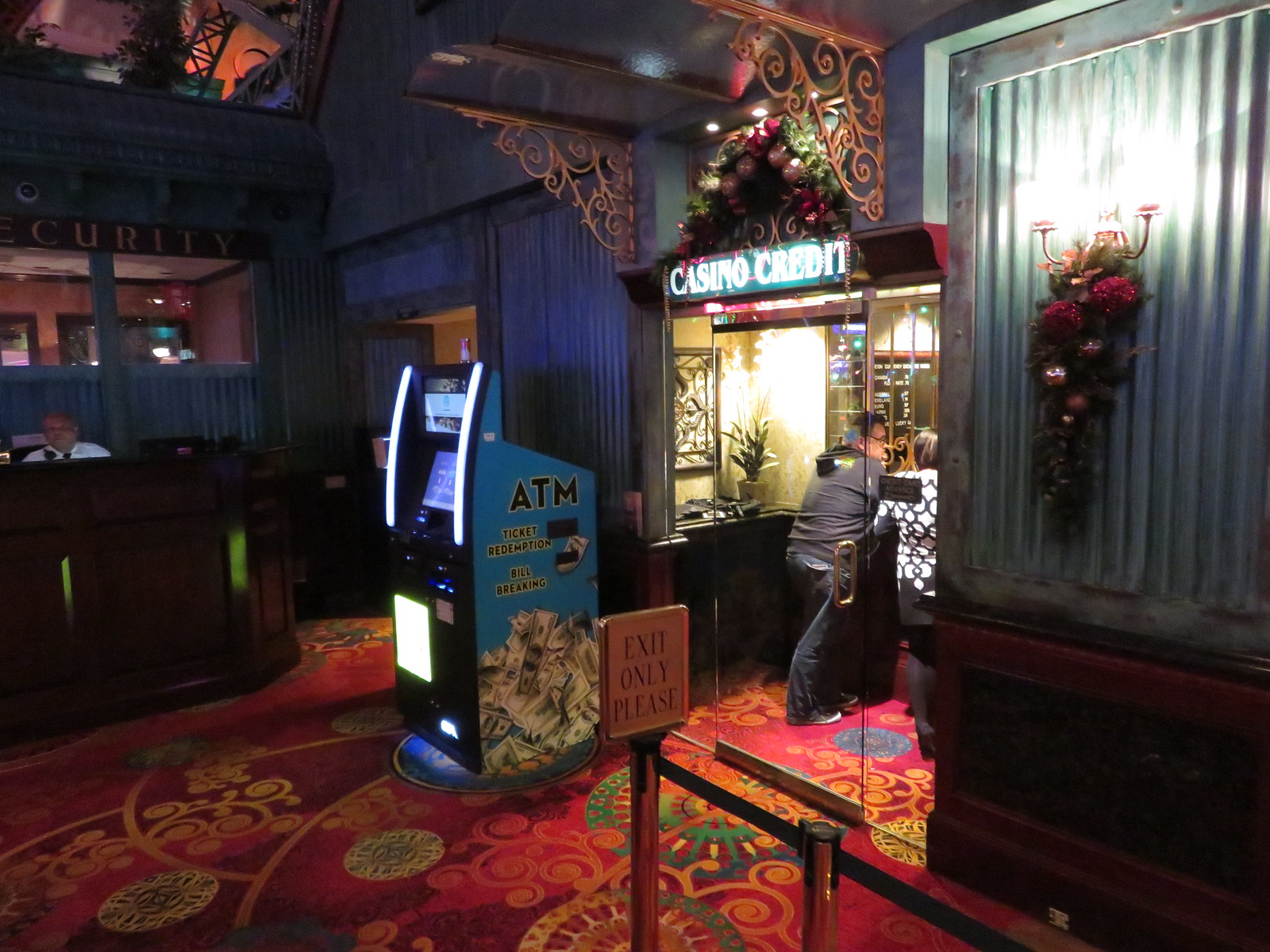This photograph captures the interior of a casino illuminated with soft lighting, highlighting various features and activity within the scene. Dominating the right side of the image is a glass-enclosed booth marked "Casino Credit" in bright white lights, which contrasts sharply with the otherwise subdued lighting. Inside, a man dressed in a black hooded jacket and black pants, alongside a woman wearing black pants and a white and black top, are conversing with someone behind the counter. Adjacent to this booth, an ATM machine stands prominently, likely a popular spot for patrons. Below, a velvet rope indicates the exit with a sign that reads "exit only please." To the left of the ATM, there is a small enclosed area resembling a café or a security checkpoint, where a person dressed in white, possibly a security guard, is seated. The carpet, resonating with an older, opulent casino style, features an intricate Oriental design in red hues reminiscent of the 1980s and 90s casinos. The overall ambiance of the photo combines elements of retro decor with the lively, transactional atmosphere typical of a casino environment.